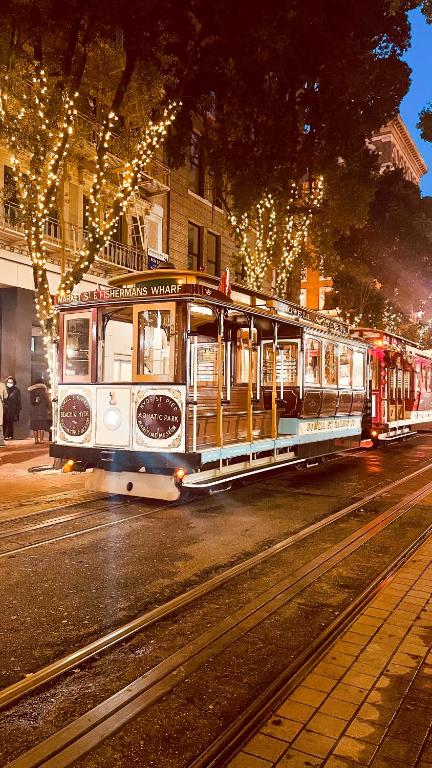The image depicts a street scene with a trolley cart, characteristic of San Francisco’s cable cars, prominently moving at an angle toward the left. The trolley consists of two carts; the front cart, primarily colored gold and white, features a white front with brown circles and a distinctive wood-colored door above which is a dark brown door. The second cart appears red and white in color. The trolley is traveling along the rails embedded in a concrete street, which looks slightly wet towards the end.

In the bottom right corner, part of the sidewalk is visible. To the left of the trolley cart, a tree adorned with Christmas lights stands by the roadside, and midway down the trolley’s side, another similarly lit tree is present. Behind these trees, a light brown building with balconies is situated on the left side of the image. At the base of this building, near the trolley cart, two people are seen standing on the sidewalk. The scene has an overall festive atmosphere due to the holiday lights, and the background transitions to a darker tone with a hint of a light blue sky visible in the top right corner. The trolley bears the title "Fisherman's Wharf," adding to the iconic San Francisco setting.